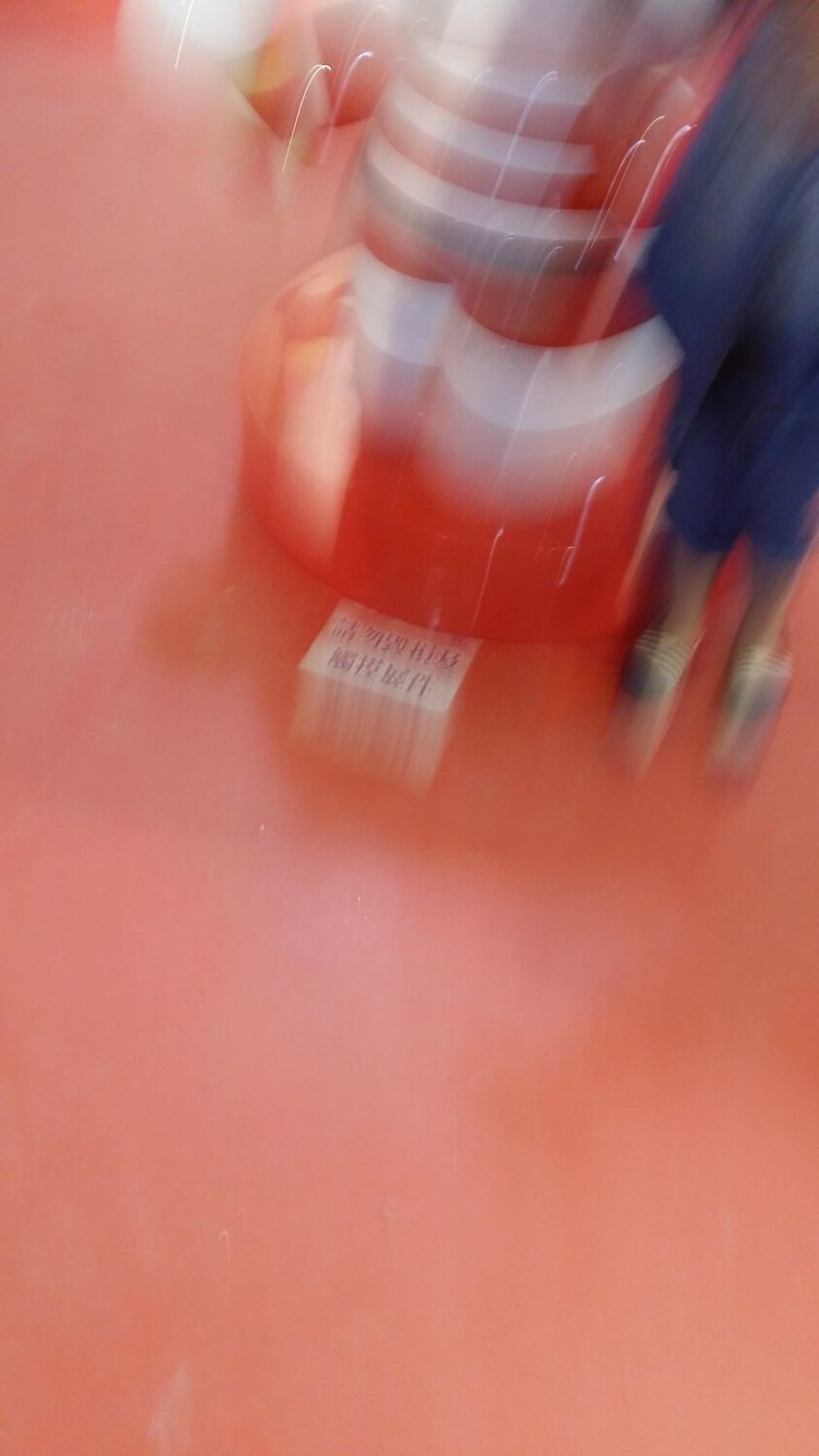This is a very blurry photograph primarily showcasing a pink or red flooring that dominates the image's lower half and left side. Toward the top right, a person is standing. This individual is dressed in a blue outfit, which could be either a dress or a pant set, and is wearing beige or possibly black sandals with white and black straps, revealing their bare legs. Adjacent to the person is a large, indistinguishable object that has notable red and white features; it might be a towering plastic item, a character with feet, or even a robot or mannequin with blocky arms. There is also a white sign with Japanese lettering located near the object on the floor. Although the exact setting is unclear due to the blurriness, light is streaming from above, adding some illumination to the scene.